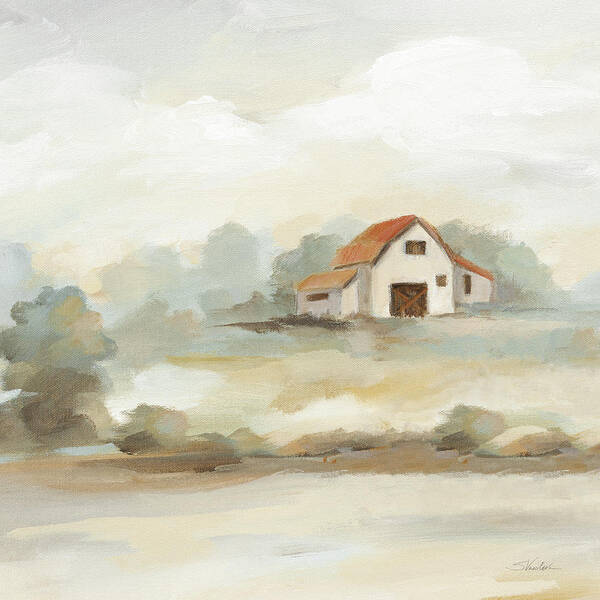This detailed square-format watercolor painting depicts a serene farm setting, featuring a prominent white barn with a high-peaked, red-shingled, gabled roof. The barn is beige at the base with greenish-gray trees behind it, blending seamlessly into lush green grass and areas of soil and rocks. The barn’s doors are located where a double garage door might be, presenting a wide, dark brown wooden opening, while above, a single window suggests a hayloft. Flanking the main structure are two smaller shed-like sections, the one on the left being lower and the one on the right slightly higher. The foreground includes subtle beige and gray tones with a horizontal line of rocks and plants stretching across the scene. Overhead, soft brushstrokes depict white, puffy clouds against a tranquil sky. The entire artwork is executed in a gentle wash of colors, emphasizing the fluidity and softness typical of watercolor painting.